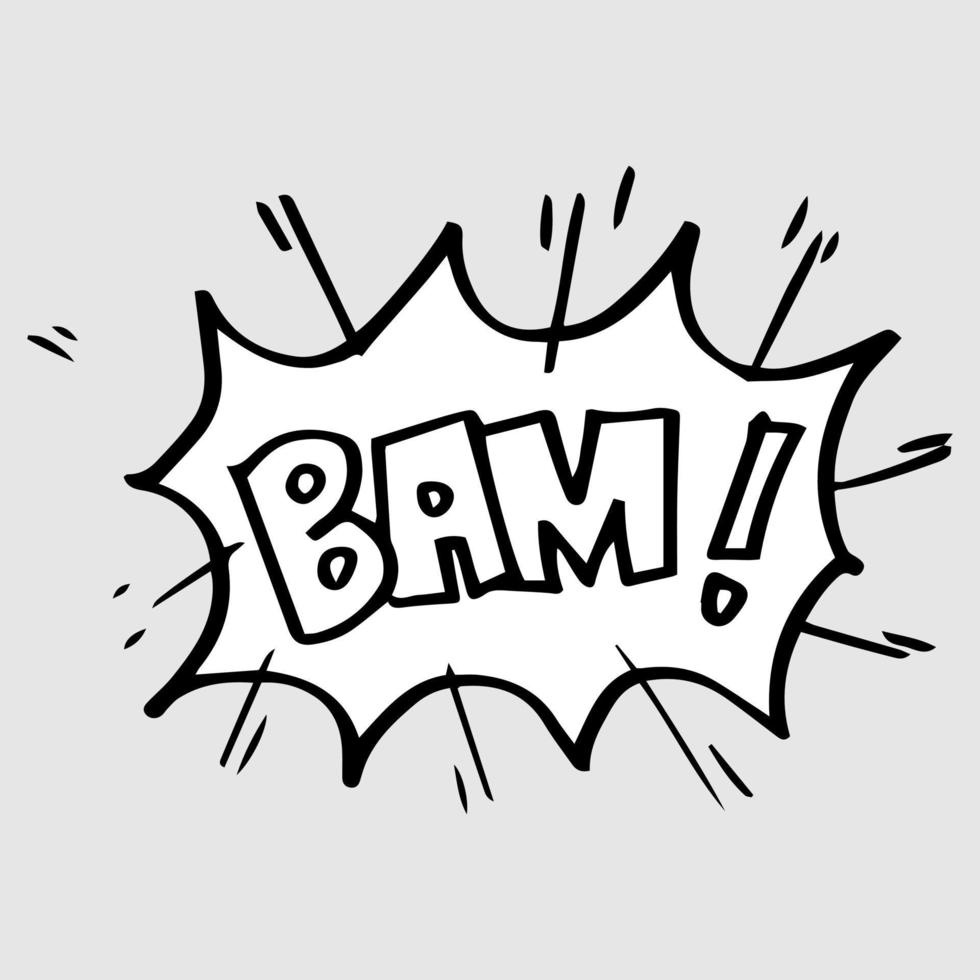The image is a cartoon-like drawing with a soft gray background featuring swirling black lines, resembling the energetic strokes of a marker. The central focus is a large, explosive text bubble with a black outline, forming spiky, dynamic edges. Inside this bubble, the background is white, providing a stark contrast to the bold, black letters outlined in black, with white centers. The letters spell out "BAM!" in heavy, capitalized typography, complete with an exclamation mark, creating a powerful and impactful visual effect. Black lines radiate outward from the bubble, emphasizing the explosive nature of the text.